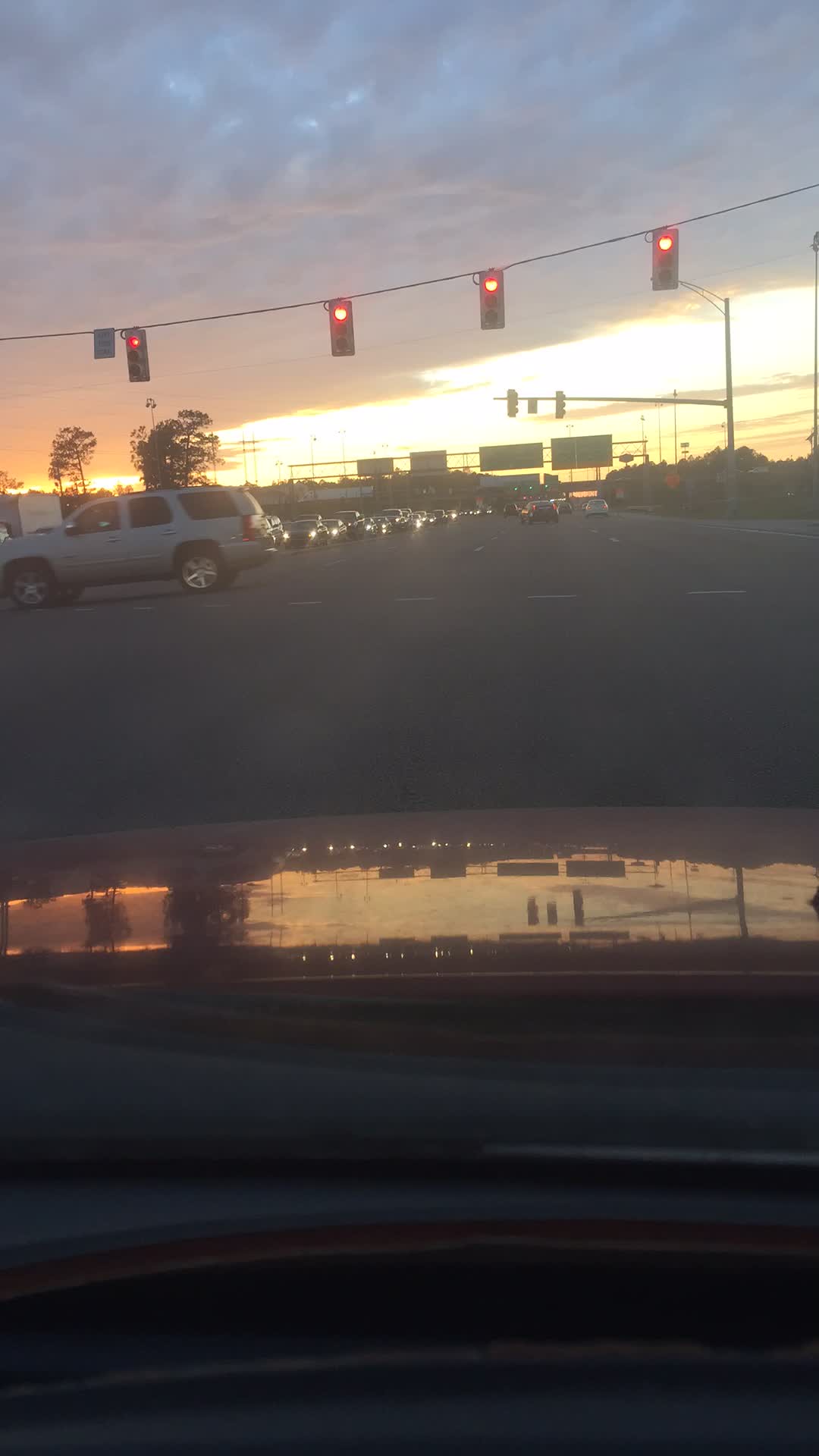The image captures a scene from inside a car at dusk, framed vertically from top to bottom. The photo was taken through the windshield, revealing the car’s dark dashboard and hood, which reflects the sky. The car is stopped at a large, busy intersection with six lanes of traffic. Four red traffic lights hang from a black cable strung across the intersection, signaling all vehicles to stop. An SUV is seen crossing the intersection on a green light. The sky is a dramatic backdrop, filled with heavy clouds but illuminated by the last light of the setting sun. Oncoming traffic is visible across the lanes, with headlights indicating a substantial flow of vehicles. In the distance, another set of traffic lights and large metal freeway signs with four green panels can be seen. The portrayal suggests an American highway setting with a poetic mix of evening light and heavy clouds.